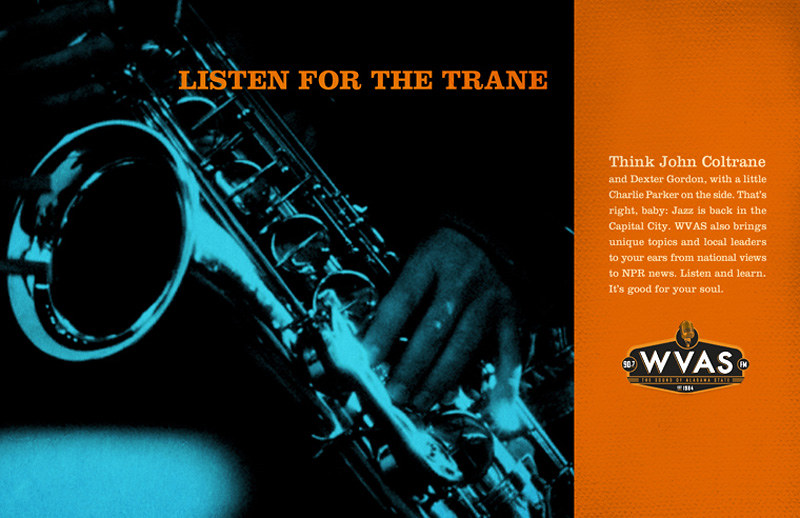The image is a horizontally aligned rectangle, divided into two distinct sections. On the left, a square segment features a close-up, black-and-white image of a hand playing a diagonally positioned saxophone. Orange text in all caps reads “LISTEN TO THE TRANE, LISTEN FOR THE TRAIN, T-R-A-N-E,” contrasting sharply against the predominantly dark background. On the right, a vertical rectangular section presents an orange backdrop with white text at its center. The message reads, "Think John Coltrane and Dexter Gordon with a little Charlie Parker on the side. That's right baby, jazz is back in the capital city. WVAS also brings unique topics and local leaders to your ears from national views to NPR news. Listen and learn, it's good for your soul." Below this text, a white logo displays the call letters "WVAS." This composition resembles a flyer or advertisement for a jazz radio station, engaging viewers with its striking visual and textual elements.